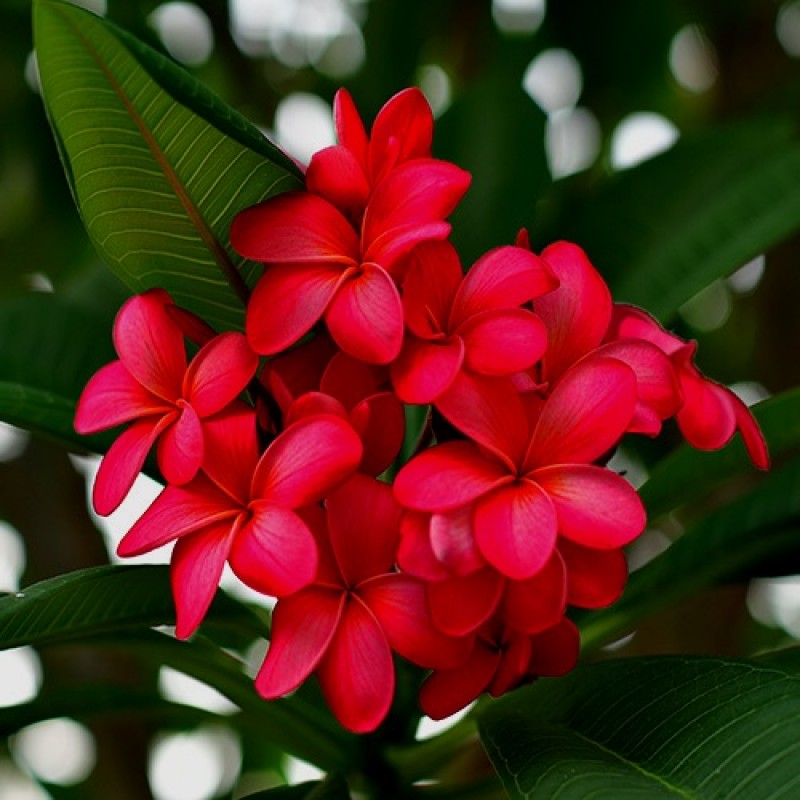This square photograph, taken outdoors, features a close-up of a vibrant cluster of red Plumeria flowers at the center. The cluster comprises about a dozen flowers, each with five slightly curled, overlapping petals that flare out gracefully at the edges. The petals exhibit a rich reddish-pink hue and appear thick and almost leathery in texture. Surrounding the flowers are several large, vivid green leaves that branch out, particularly to the top left and the bottom right of the image. The leaves are thick and dark, enhancing the tropical feel of the scene. The background is intentionally blurred, showcasing a mix of whites and greens likely indicating more plants and diffused light from the sky. The contrast between the sharply focused flowers and leaves and the soft, indistinct backdrop accentuates the lush, detailed beauty of the Plumeria in this photograph.